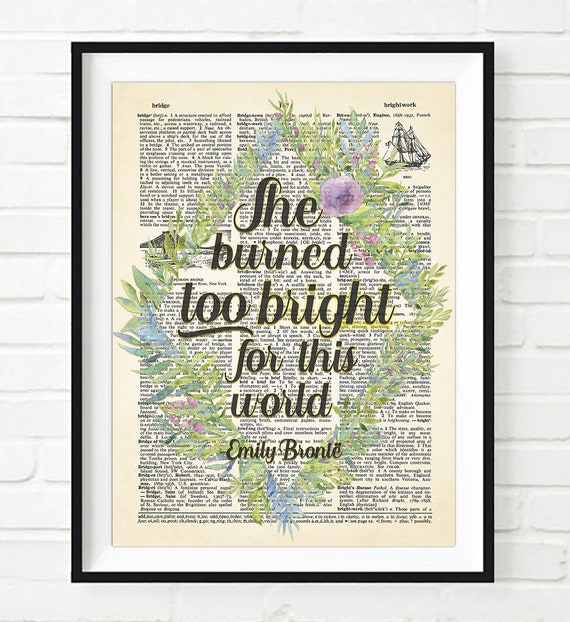This image, framed in a sleek black border with a white mat, hangs against a pristine white brick wall. The central artwork resembles a page from an old newspaper, characterized by three vertical columns of unidentifiable black text on yellowed paper. The top right corner features an intricately illustrated ship with full sails. Additionally, a smaller, stylized illustration of a bridge appears in the left column. Overlaying the text, a diamond shape is formed by green plant stems adorned with vibrant purple and blue flowers. Within this floral diamond, in elegant, dark green cursive script, the poignant quote "She burned too bright for this world" is prominently displayed, attributed to Emily Bronte beneath it. The juxtaposition of vivid natural elements and classic typography against the monochrome frame creates a visually captivating piece.